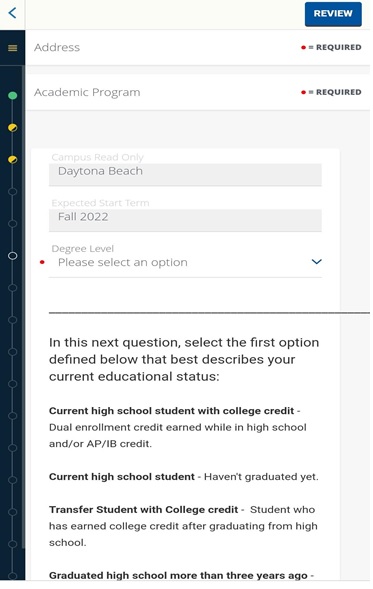In the top right corner of the image, a blue box contains the word "REVIEW" in all capital letters. Moving to the left side, there is a long vertical blue box. At the top of this vertical box, a small gray box is placed, followed by a green circle and two yellow circles further down.

In the central area of the image, the word "ADDRESS" is prominently displayed, with a red circle and the word "REQUIRED" next to it. Below "ADDRESS," the text "ACADEMIC PROGRAM" appears, accompanied by another red circle and the word "REQUIRED." Approximately three inches below "ACADEMIC PROGRAM," a search bar contains the text "DAYTONA BEACH." Below this search bar, another search bar displays "FALL 2022."

Underneath, the section labeled "DEGREE LEVEL" includes a red circle and the text "PLEASE SELECT AN OPTION," along with an arrow icon indicating the option to click and select. A long horizontal line separates this area from the following section.

The next section begins with a prompt: "Select the first option defined below that describes your current educational status." Listed in bold black text are the options:
- CURRENT HIGH SCHOOL STUDENT WITH COLLEGE CREDIT
- CURRENT HIGH SCHOOL STUDENT
- TRANSFER STUDENT WITH COLLEGE CREDIT
- GRADUATED HIGH SCHOOL MORE THAN THREE YEARS AGO